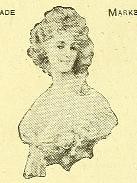This image is a small, intricate drawing or print—resembling perhaps an old-fashioned stamp or an illustration from an antique book cover—featuring a young woman from a bygone era, possibly the 1800s to early 1900s. The woman's figure, depicted from the bust up, stands central against a yellow background. She dons an elaborate and elegant dress, characteristic of royalty, with a soft, white, blouse-like upper garment. Her long hair is styled in a sophisticated manner, and she gazes thoughtfully over her left shoulder. The contour of her face and body is rendered in black and white, providing a stark contrast to the yellow background. The image also contains partial textual elements at the top; the letters "A-D-E" are visible on the left with "M-A-R-K-E" on the right, possibly suggesting the fragments of some form of titling or mark.